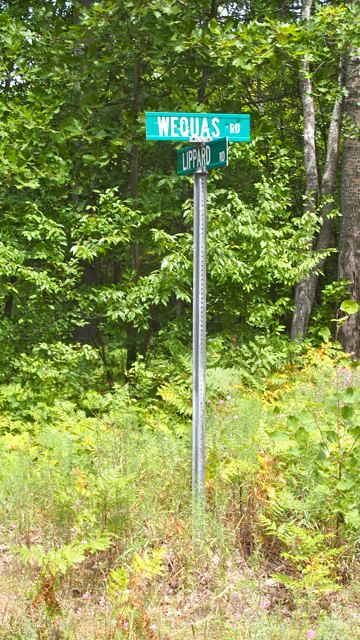A vibrant, real-life image captures a metal post at the junction of two streets, highlighted by green street signs with white text. One sign, facing the camera directly, reads "We Cross Road," while the perpendicular sign at a steep angle appears to read "Lipard Road." They both feature a dark green background and white lettering. Surrounding the metal post is a wild, unkempt area with overgrown weeds, dry grass, and spiny plants hinting at a recent dry spell. The scene is bright and bathed in sunlight, illustrating the need for water among the light green plants. In the backdrop, a mix of greenery flourishes, including trees with light gray bark and darker-leaved trees, creating a juxtaposition between the street sign and the natural environment. The overall setting emphasizes the rural and untamed nature of the location, bathed in the clear daylight.